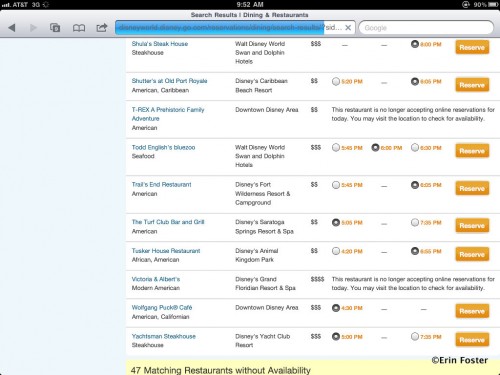This image is a slightly blurry screenshot taken from an Apple device, likely an iPhone or iPad, evident from the display at the top showing the service provider, reception, time, and battery percentage. The screenshot captures a browser window, presumably Safari, with nine open tabs. The visible webpage details search results for dining and restaurants. While the URL is unclear, the top of the page states "Search Results: Dining and Restaurants." 

The main content displays a list of restaurants, each entry providing the restaurant's name, location, and price range, indicated by dollar signs. The page also indicates the availability of reservations with an orange "Reserve" button next to each listing. Notably, the search resulted in 47 restaurants without available reservations at that moment. 

The screenshot includes a watermark in the bottom right corner that reads "Aaron Foster," suggesting they are the individual who captured the image.